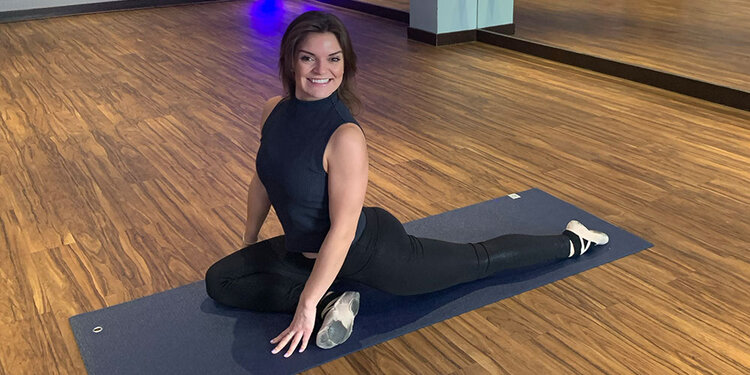This is a detailed photograph of a white Caucasian woman with brown hair and brown eyes, performing a yoga pose on a light brown wooden studio floor. She has long brown hair tied back, extending past her shoulders. She’s positioned on a blue yoga mat, angled at 45 degrees to the camera. 

The woman is dressed in tight black pants, a light blue tank top, and white shoes with black stripes. She is in a stretch with her right leg bent forward, the sole facing the camera, and her left leg extended backward, the top of the foot resting on the floor. Her arms are resting on the mat in front of her, with her back arched, and she is looking at the camera, smiling enthusiastically.

The studio’s interior features mirrors on the right side of the frame, black baseboards beneath them, and a noticeable deep purple reflection of light at the far end of the studio, near the top center-left of the frame. There are no writings or additional elements in the image, and the ambient setting suggests a modern-day photograph.